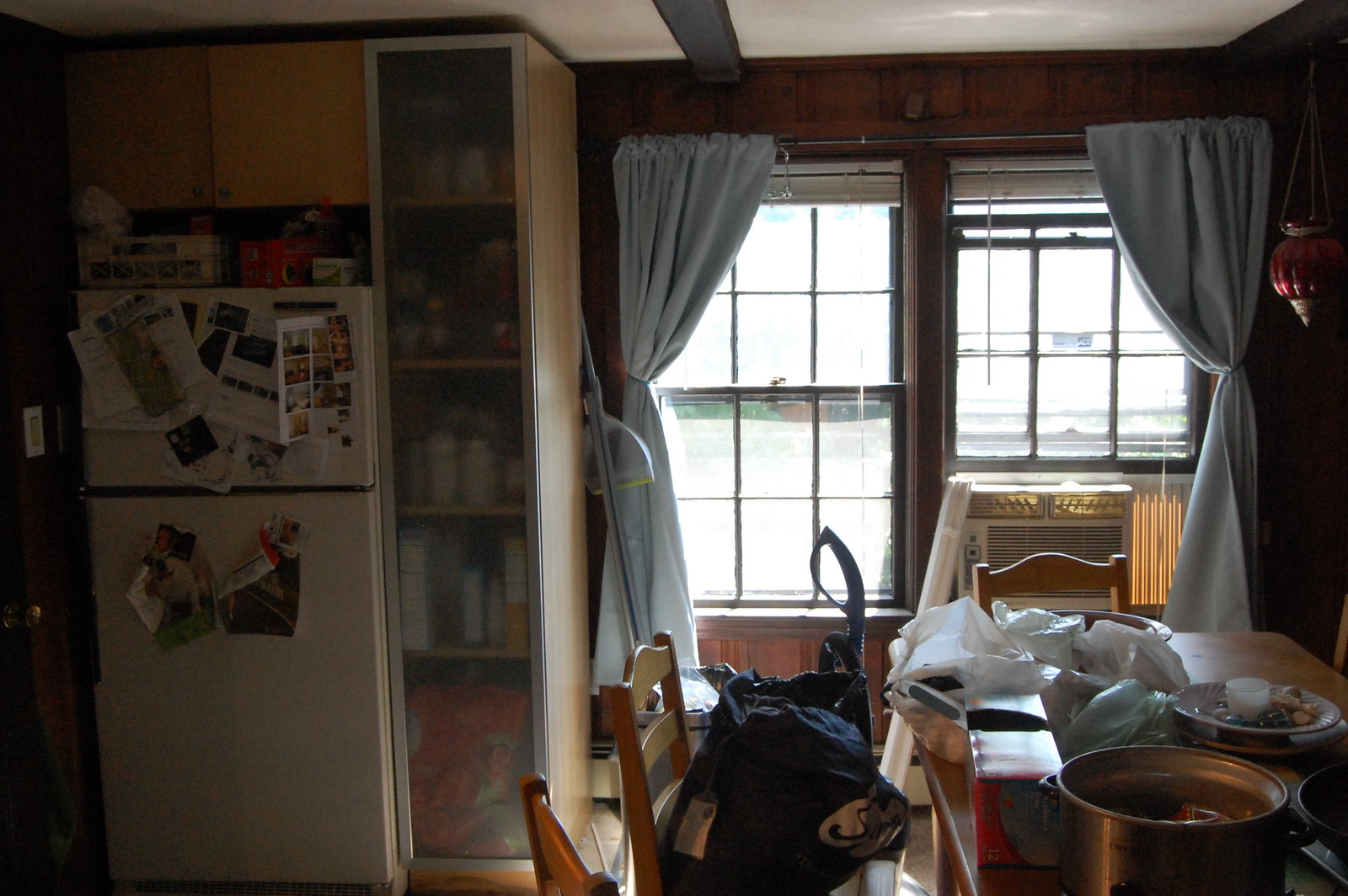In this first-person POV image of a dining and kitchen area, a wooden dining table occupies the central focus. Seen from the perspective of the image taker, the table features three chairs: two on the left-hand side and one at the head of the table furthest from the viewer. Behind this chair, a heater or air conditioner is installed under a window, which is flanked by greyish curtains drawn open to let sunlight pour in, creating a glare on the window’s reflection. 

The gridded windows feature two panes that slide up to open, each divided into six smaller sections (two columns and three rows). To the left of these windows stands a tall pantry cabinet with a frosted glass door, concealing five internal shelves— the bottom shelf being the largest. Adjacent to this pantry unit, a refrigerator stretches from floor to ceiling. The fridge's design includes a larger lower compartment and a smaller upper freezer section, both adorned with various papers and photos. Notably, a photo of a dog is attached near the handle on the left side of the fridge door. 

On the wooden dining table, an assortment of items is scattered, including plastic bags, a wok, cling film, and a plate with miscellaneous objects that appear to be gemstones.